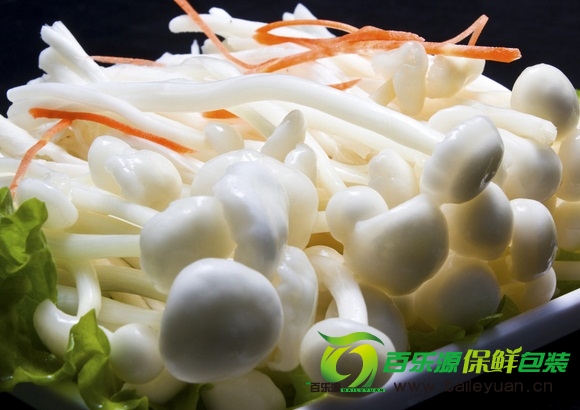This close-up photograph features a dish composed primarily of white sprouts arranged in a neat pile atop a white ceramic plate with a slight ledge. The sprouts, appearing glossy and almost mushroom-like with their cylindrical stems and mushroom-shaped heads, are accented by thin strands of shredded orange carrot. Beneath the sprouts lies a subtle bed of light green lettuce, visible along the left-hand and bottom edges of the plate. The entire arrangement is set against a stark black background, creating a striking contrast. In the bottom right corner of the image, a green and yellow brand symbol is prominently displayed, accompanied by a series of Japanese or Chinese kanji characters written beneath it, followed by what appears to be a web address in dark gray text, "www.valley1.cn."